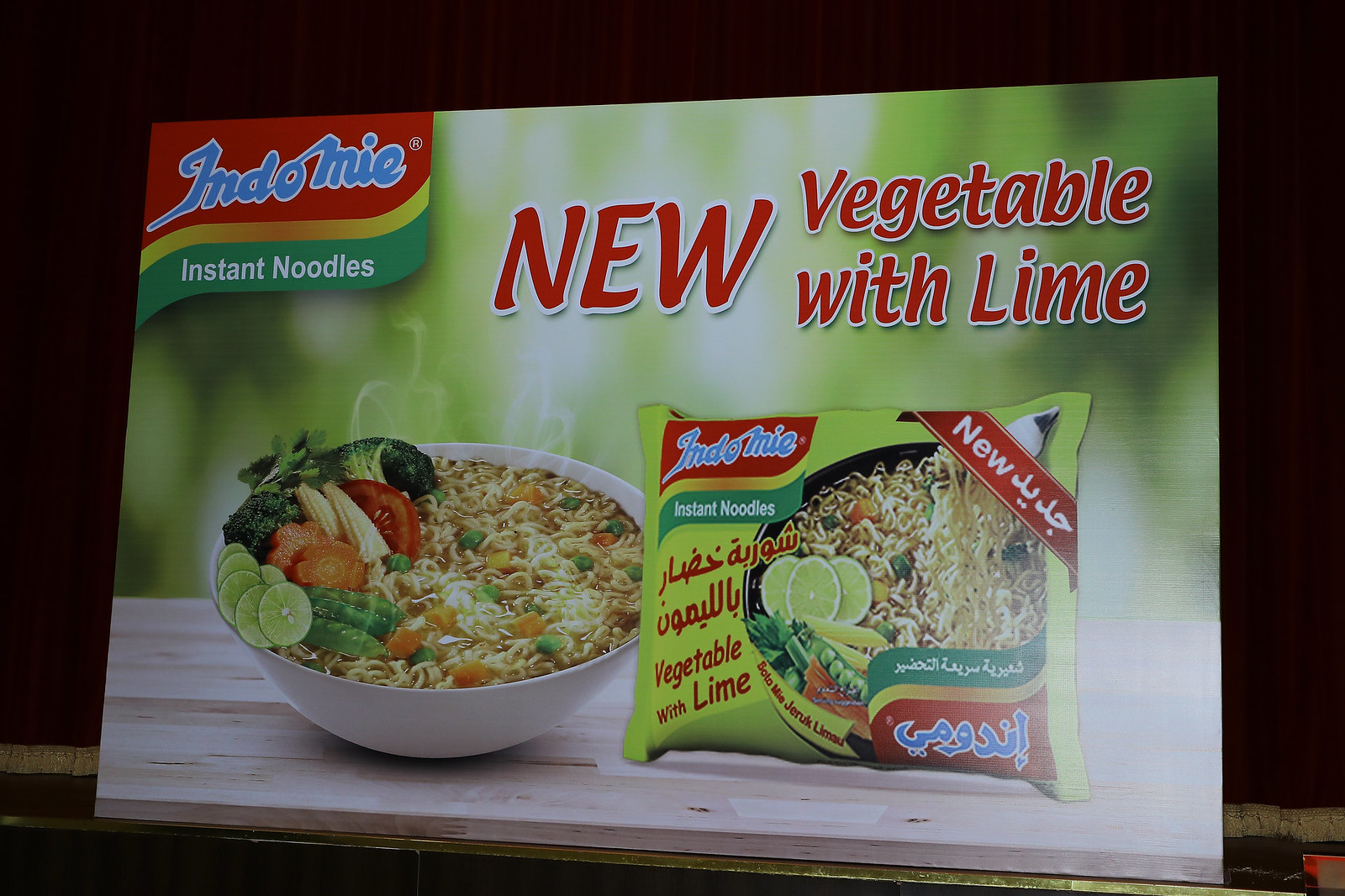This advertisement photograph showcases a promotional banner for Indomie instant noodles, specifically highlighting their new "Vegetable with Lime" flavor. The banner is prominently displayed on a wooden slab and features the Indomie logo in the top left corner. To the right of the logo, bold red letters with a white outline announce "new vegetable with lime." Below this text, the packaging for the lime-flavored noodles is depicted, displaying a bowl of noodles brimming with lime slices, peas, carrots, baby corn, broccoli, and other vegetables.

Adjacent to the packaging, on the left side, is a steaming bowl of the product showcasing a colorful assortment of ingredients. This includes neatly arranged chopped carrots, baby corn, limes, peas, broccoli, and various smaller vegetables. The steam rising from the bowl underscores the freshly cooked appeal of the noodles. The entire scene is set against a wooden surface, suggesting a rustic dining setting.

The background of the banner appears to have a dark or greenish hue, possibly resembling out-of-focus leaves or branches, adding a natural and fresh ambiance to the advertisement. The setup of the banner gives the impression of it being propped up or leaning slightly against this dark backdrop, emphasizing its presence while maintaining focus on the vibrant imagery of the noodle dish.